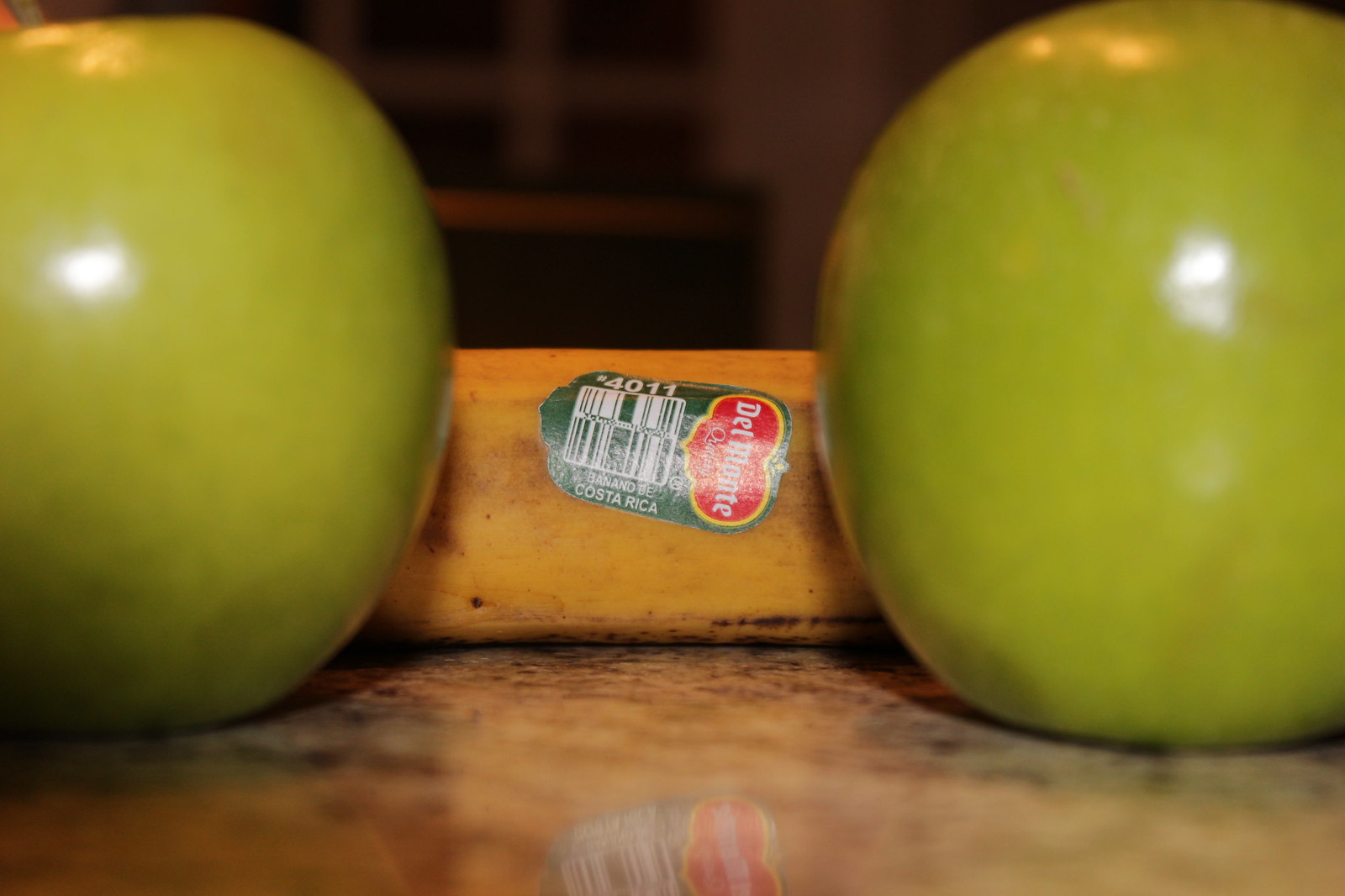In this landscape-oriented image, two prominent green apples occupy the left and right thirds of the frame, almost filling the scene from top to bottom. Nestled between the apples, partially concealed by their shiny green exteriors, lies a ripe Del Monte banana. The focal point of the image is undeniably the banana, highlighted by its distinct label. The label features a red background circled by a yellow band, showcasing the Del Monte brand, the number 4011, and its origin—Costa Rica. The foreground table surface, though initially out of focus, gains clarity closer to the banana, revealing a potential brown marble or quartz texture. The visual emphasis on the banana against the contrasting shiny green apples and the textured table surface creates a striking and detailed composition.